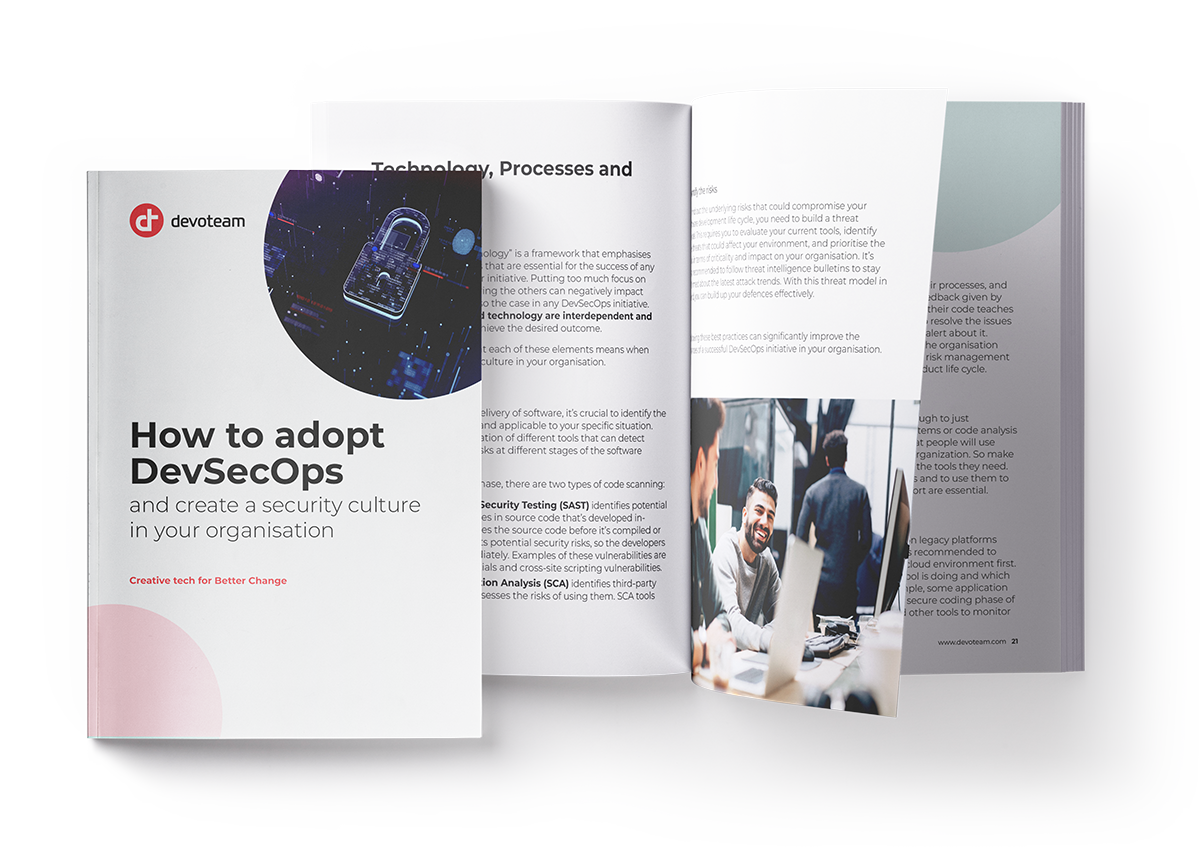The image depicts a product concept for a business book about cybersecurity. The cover, positioned on the left side of the image, features a digitalized, glowing blue lock against a dark blue background in the top right corner, symbolizing cybersecurity. In the top left corner, the cover displays the Devoteam logo. Centered prominently, the title reads: "How to Adopt DevSecOps and Create a Security Culture in Your Organization," followed by a tagline in red letters: "Creative Tech for Better Change." The right side of the image shows a rendering of the book opened, with a page turning from right to left. The open pages feature black text on a white background, and one of the pages includes a photo at the bottom half, depicting a man at a computer smiling at a colleague behind him. The image provides a comprehensive view of both the book cover and its interior layout.